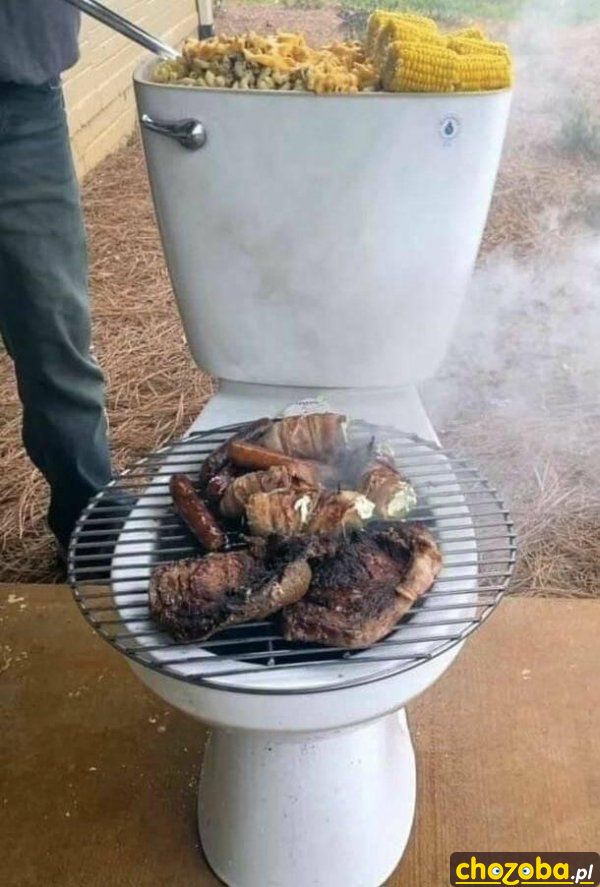This vertically oriented image features an unusual makeshift grill crafted from a classic white porcelain toilet, prominently placed in the center. The toilet stands on a brown, tan-tiled floor inside a house, transitioning to carpet where a man's leg in blue jeans and part of his torso is visible to the left side of the image. The toilet bowl has been repurposed with a silver grate placed over it, sizzling with an assortment of meats including steak, possibly lobster tails, and sausage, along with shrimp. Smoke billows from the grill, emphasizing its active use. The toilet tank, with its lid removed, contains vegetables such as corn on the cob, macaroni, and possibly crab meat. The tank also emits smoke, indicating ongoing cooking. Despite the indoor setting, references to dead grass and cement suggest a possible outdoor environment mingled in the description. In the bottom right corner, the term “ZOBA” is prominently displayed, resembling a clickable link but without a full URL, hinting at the peculiar nature of this toilet-turned-grill.